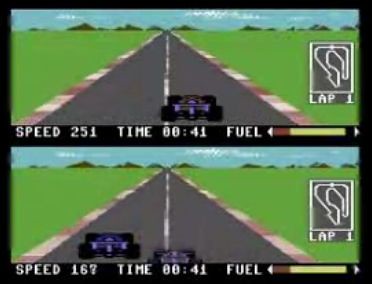This is a screenshot from a vintage two-player racing video game. The screen is divided into two sections, one for each player, with a thick black border around and between them. Both screens feature a background of a blue-teal sky with white fluffy clouds and green grass flanking a basic gray asphalt road. The road has alternating red and white stripes along either side, evoking a race track aesthetic.

In the top section of the screen, the player-controlled vehicle is a blue race car with big wheels and a small body, positioned in the right lane. The interface shows critical data: a speed of 251, a time of 41 seconds, and a fuel gauge indicating near full fuel with a gradient from red to green. The top right of this section also displays 'Lap 1' and the car's position on a mini-map.

The bottom section mirrors the top but with a slight difference in vehicle placement. Here, the car is in the left lane, showing the front end of the player one's car still in the right lane. The data indicates a lower speed of 167, the same time of 41 seconds, and a corresponding fuel gauge. Additionally, the bottom right shows the mini-map with the car's location on the track.